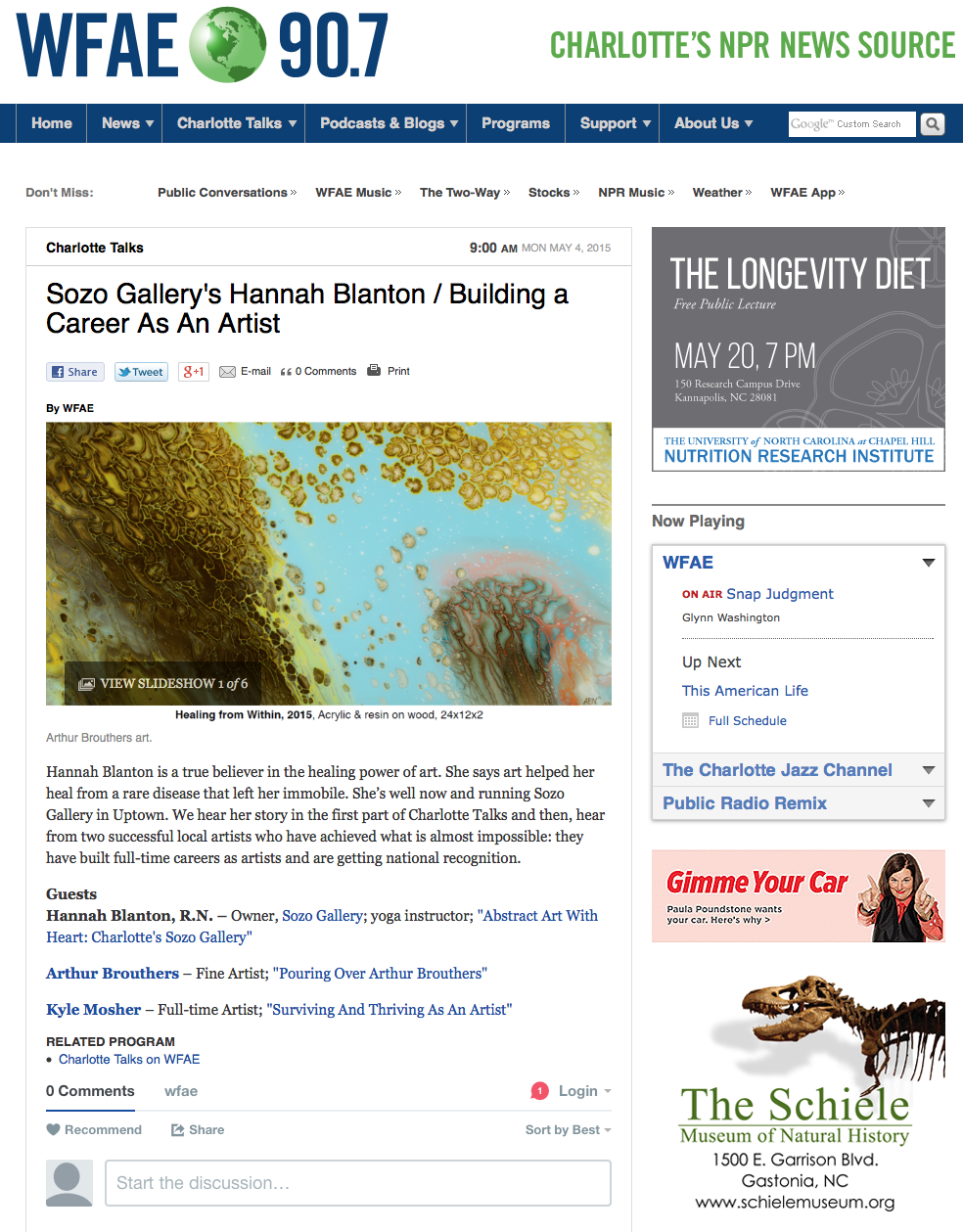The image is a color, portrait-oriented screenshot of a website being browsed on a laptop. The website is for WFAE 90.7, a radio station. At the top of the page, the station's name is prominently displayed in blue lettering alongside a logo depicting a blue globe with North America at its center. In the top right corner, the text reads, "Charlotte's NPR News Source," with NPR standing for National Public Radio.

The website's navigation bar includes several tabs: Home, News, Charlotte Talks, Podcasts and Vlogs, Programs, Support, and About Us. 

In the center of the page, there is a featured article titled "Sozo Gallery's Hannah Blanton: Building a Career as an Artist." The article highlights Hannah Blanton, who credits art with helping her recover from a rare disease that left her immobile. Now fully healed, she runs Sozo Gallery in Uptown Charlotte. The article also teases an interview with Hannah Blanton on "Charlotte Talks" and mentions two successful local artists who have achieved national recognition for their full-time art careers.

Below the article, there is an option for readers to add comments, and along the far right side of the page, a series of advertisements are displayed.